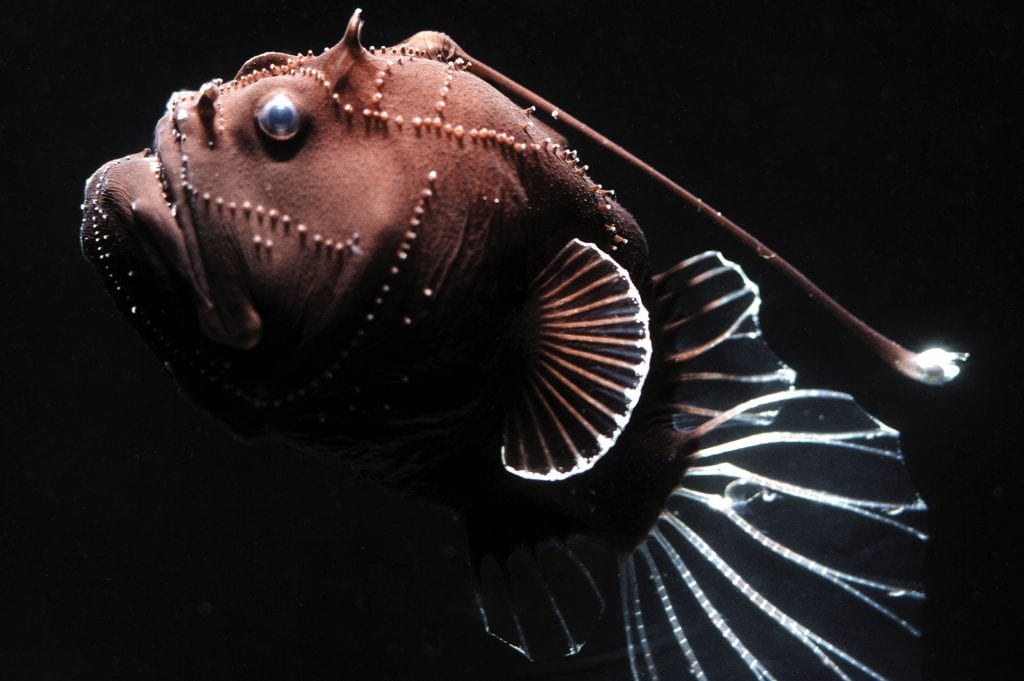This underwater photographic image features a distinctive deep-water fish captured against a solid black background, giving it a striking appearance. The fish is diagonally positioned from the bottom right to the top left, showcasing its elongated body and pronounced snout. Its eyes are large and boat-like, enhancing its mysterious deep-sea allure. The fish's head is adorned with a myriad of small brown and white dots, adding intricate details to its overall appearance. A notable feature is its long antenna, extending in a downward diagonal towards the bottom right corner, ending in a white dot.

The fish's tail is black with white stripes, while its fin exhibits a vivid pattern of black and orange stripes bordered by white, resembling the elegant folds of a hand fan. This unique combination of colors and patterns gives the creature a somewhat fantastical and unreal aspect, reminiscent of beaded designs or handcrafted art. The scene is devoid of any textual elements, allowing the viewer to fully immerse in the visual intricacies of this underwater marvel.